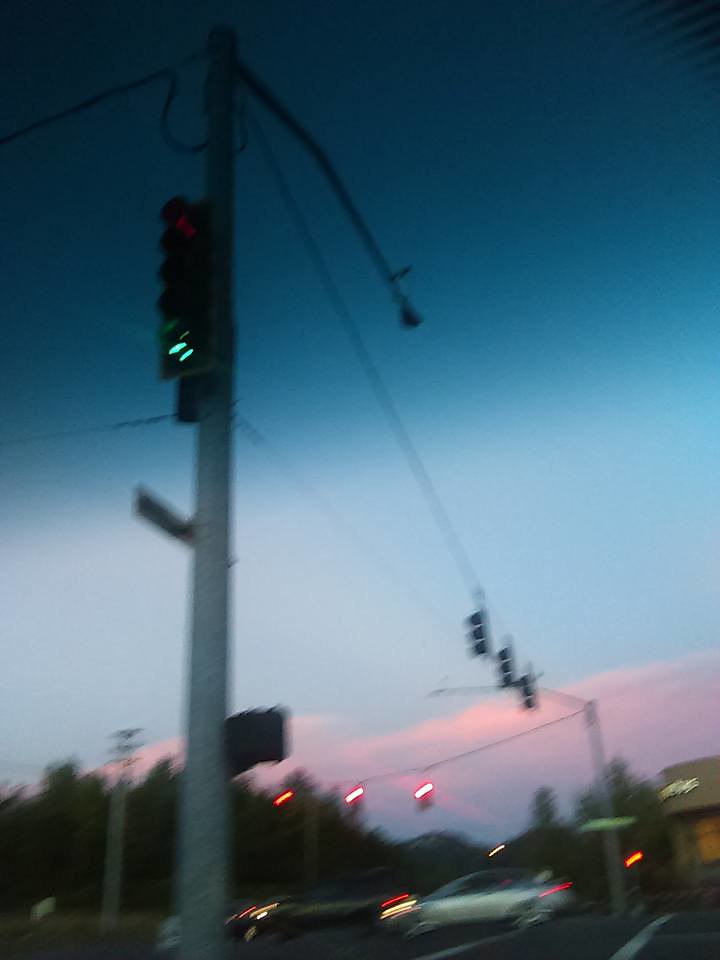A slightly blurry photo taken, possibly with a camera phone, captures a road intersection at dusk, just before evening. In the foreground, one corner of the intersection is visible. A traffic light is prominently featured; the red light shines at the top, with the green light below it, consistent with standard traffic signal arrangement. Beneath the traffic light, there's a street sign, and directly below that is the pedestrian signal indicating when it is safe to cross.

Across the intersection, all visible traffic lights are red. The bottom right corner of the image shows part of a building, though the text on it is unreadable due to the blurriness. It might be some kind of restaurant. Two vehicles are driving through the intersection from right to left—a silver car followed by what seems to be a dark or black SUV. The perspective of the image suggests it was taken from one corner of the intersection, giving a view of the opposite end and the right side but not the left side of the intersection.